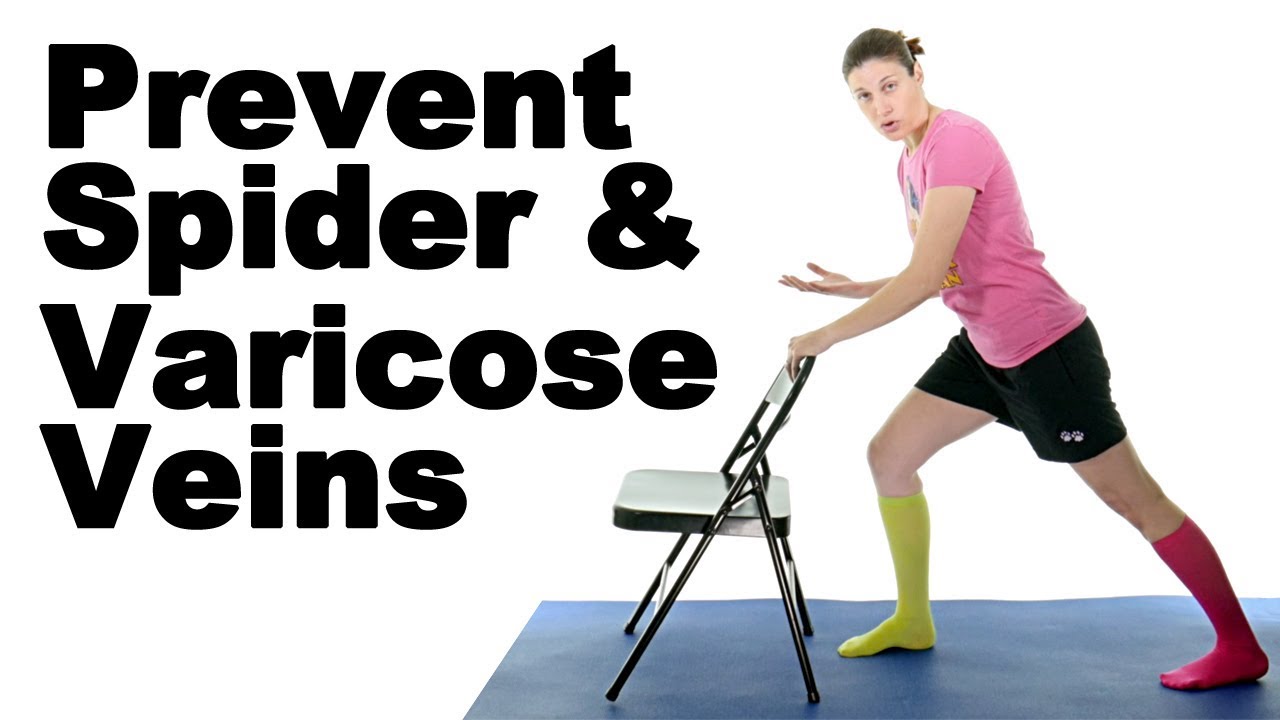In a horizontally oriented photo with a white background, a woman is pictured standing on a blue exercise mat, appearing to perform a lunge or stretch behind a black, shiny folding chair. She is facing slightly to the left, with her right leg forward and her left leg back, and is using one hand to support herself on the top of the chair. She is dressed in a pink graphic tee with an unseen design, black shorts adorned with small white paw prints, and mismatched knee-high socks—one green and one pink (or yellow and red, as variants suggest). Her hair is medium-length, brown, and styled into a ponytail or bun. Prominently displayed in bold, black Helvetica text on the upper left of the image is the phrase "Prevent spider and varicose veins," which suggests that her workout is focused on leg health.